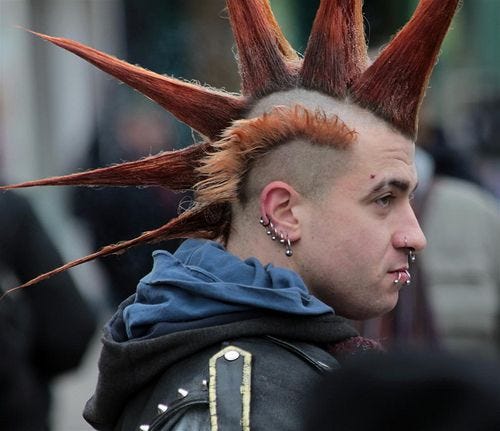In the image, there is a Caucasian man with a striking and unconventional hairstyle. He has a spiky orange mohawk that extends in a row of six large, triangular spikes, reminiscent of a T-Rex. The rest of his head is shaved, except for an orange fringe over his ear. His ear is adorned with multiple silver hoop earrings, and his face features several piercings, including his nose and bottom lip. His black eyebrows contrast with the need for a shave. He is wearing a black leather jacket with small spikes on the shoulders, layered over a blue hoodie. The background is blurred and gray, possibly depicting other people, though they are out of focus. The photo shows him from the shoulders up, facing to the right, highlighting the intensity and detail of his unique appearance.